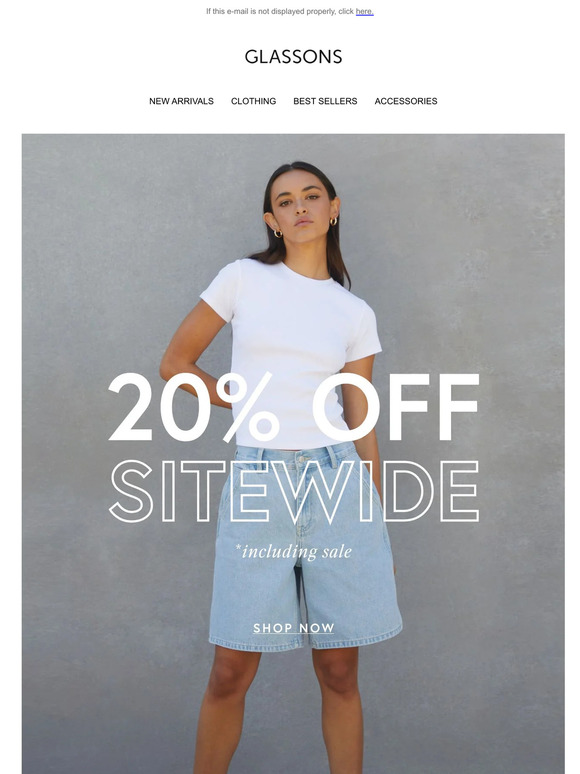The image depicts an email advertisement from Glassons. At the top, in very small print, there is a line that reads, "If this email is not displayed properly, click here," with the word "here" underlined in blue. Below this text, the company name "Glassons" is prominently displayed in black letters on a white background. 

Beneath the company name, there are four navigational options for the recipient to click on: "New Arrivals," "Clothing," "Best Sellers," and "Accessories."

The main body of the email features a large promotional image with a solid blue background. A woman is prominently displayed in the center of the image, wearing a white short-sleeved top and light blue shorts that resemble culottes, made from a jean-like material. Across the image, bold white letters announce "20% off." Directly beneath this, in white outlined letters that allow the blue background to show through, the word "sitewide" is displayed, emphasizing that the discount applies to all items. An asterisked note follows, specifying that the offer includes sale items. At the bottom of the image, a call-to-action button in white letters encourages recipients to "Shop Now."